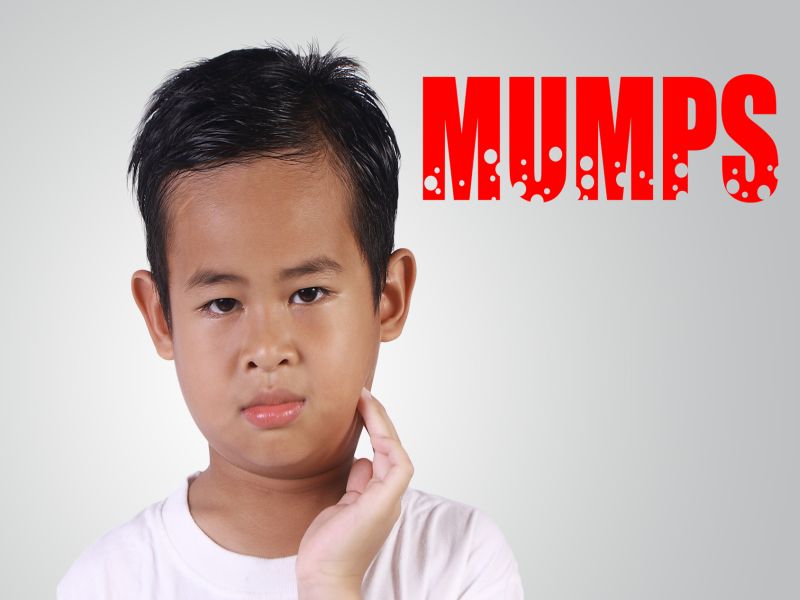The image depicts a young boy, likely around 7 or 8 years old, with short black hair and dark brown eyes, possibly of Asian or Hispanic descent. He is wearing a white T-shirt and has a hand pressed against the left side of his face, near his cheek, suggesting discomfort or swelling commonly associated with mumps. The background is a light gray color. In the upper right corner of the image, the word "MUMPS" is prominently displayed in bold red capital letters, each letter adorned with gray circles at the bottoms. The boy has a mildly crabby expression, although he doesn't appear to be in significant discomfort. The picture appears slightly stretched vertically, making his forehead seem larger than normal.